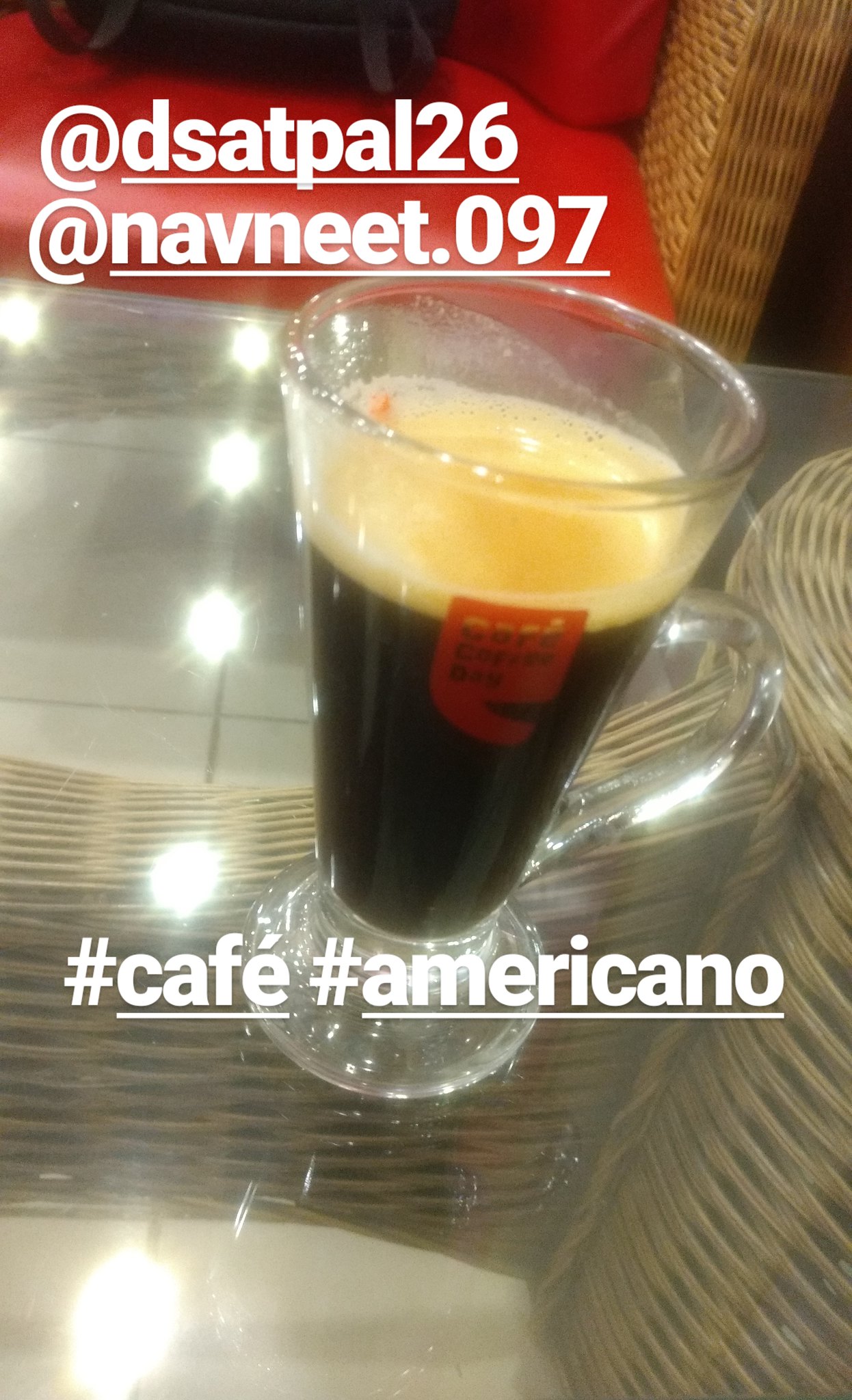The image prominently features a close-up of a small, cone-shaped glass cup perched at the center of a glass-top table, reflecting the wicker table stand beneath. This beverage, likely a shot of espresso or a similar brown liquid, showcases a layer of white foam at its top. The cup also bears a red logo, enhancing its visual appeal. Surrounding the drink, the wicker table's intricate basket material emerges, complemented by red-cushioned seating positioned towards the upper section of the image. A black or brown bag or purse rests atop one of these seats, adding a casual touch to the setting. The atmosphere suggests a cozy ambiance, likely in a restaurant, indicated further by the white on-screen text: "@dsatpal26 @navneet.097" and hashtags "#cafe" and "#americano." The color palette of the scene is a harmonious blend of red, white, brown, black, tan, and silver, contributing to the overall warm and inviting mood.